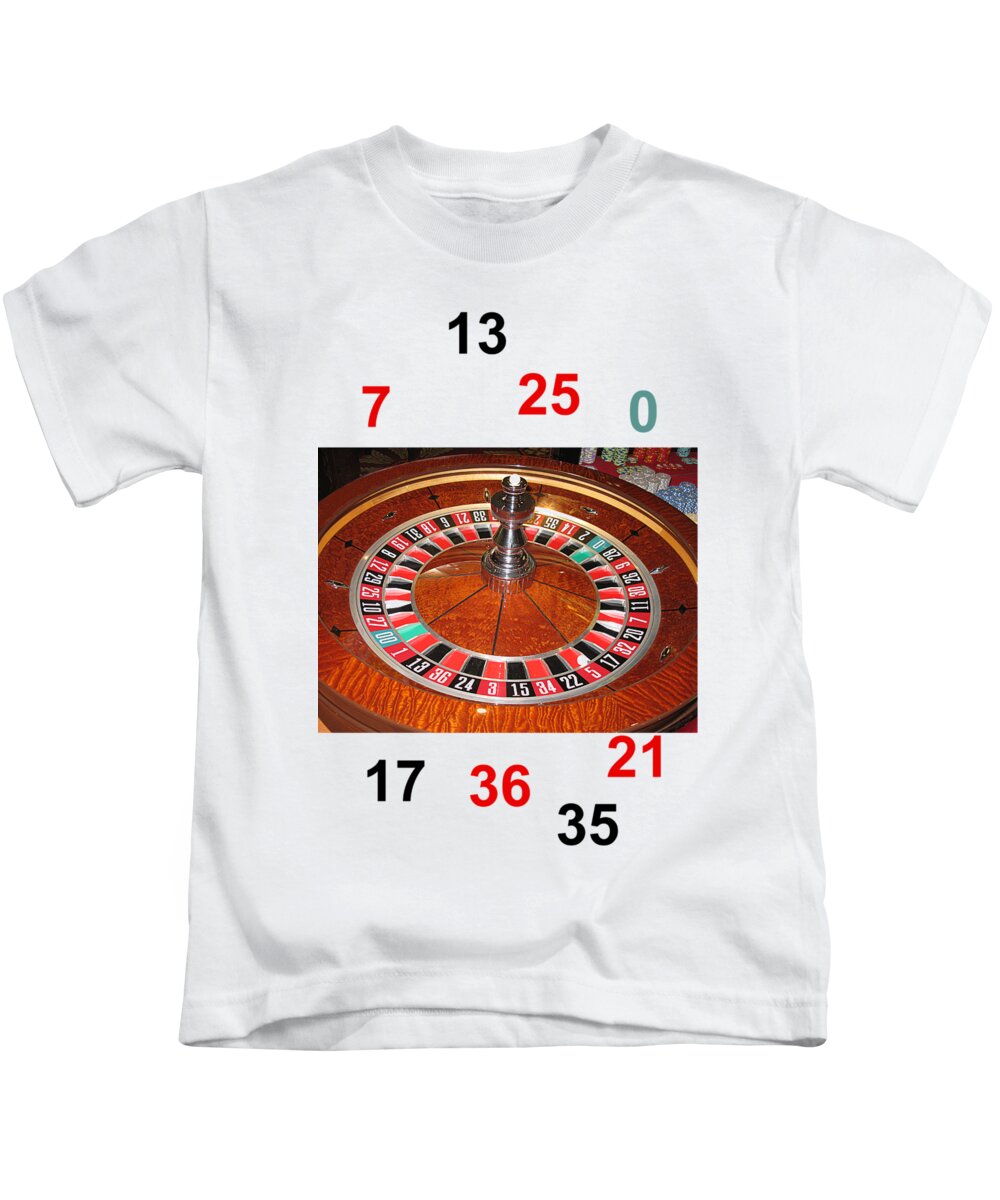This is a photograph of a basic short sleeve white t-shirt on a plain white background. The center front of the t-shirt features a large, somewhat amateurish photographic print of a wooden roulette wheel, a popular casino game. Scattered unevenly around this image are various numbers that would typically be found on a roulette wheel: 7 in red, 13 in black, 25 in red, 0 in teal green, 17 in black, 36 in red, 35 in black, and 21 in red. The randomness of the number placement and the informal appearance of the print give the impression that it might be a homemade decal.